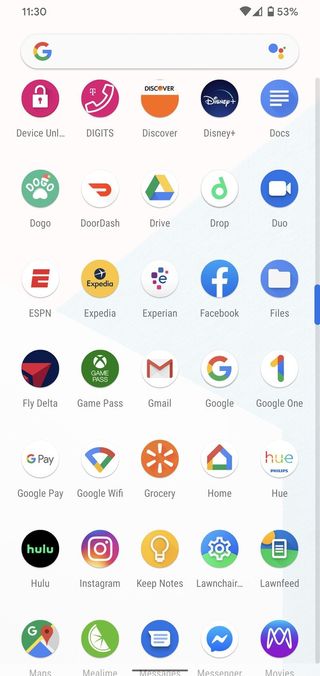A detailed and descriptive caption for the given image could be:

"This image captures a screenshot of a smartphone's home screen. At the top left corner, the current time is displayed, while the top right features a series of essential phone icons including Wi-Fi signal strength and battery level. Dominating the upper section of the screen is a large Google Search bar, complete with the distinctive 'G' logo on the left and Google's colorful circular icon on the right. Below the search bar, numerous app icons are arranged in a circular and grid-like pattern, spanning several rows. Each app icon is distinct and visually representative of the application it leads to. On the far right side of the screen, a scroll bar indicates the user's current position within the app list. There are approximately thirty apps visible on this page, organized alphabetically. The collection includes a mix of Google apps, social media platforms such as Instagram, travel tools like Expedia, among others. The structured yet comprehensive layout provides an easy navigation experience for the user."